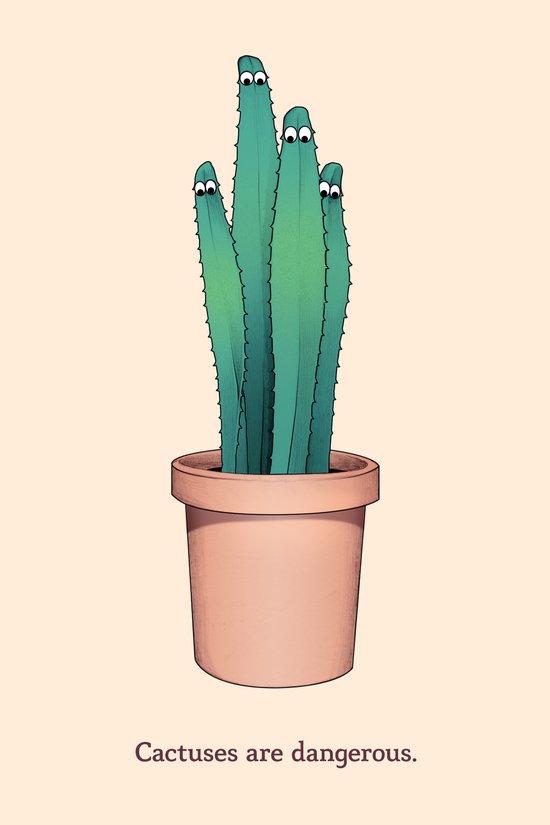Against a solid pink rectangular background, at the center of the image, stands a dark pink potted plant resembling a cactus. Four green, narrow, and tall cacti stems arise from the darker pink pot, each adorned with googly eyes at their tips, giving them a lively appearance. The eyes are white with black pupils situated at the bottom, making them seem as if they are peering downwards. The cacti's spiky, jagged edges add to their prickly and potentially dangerous look. Below the pot, a caption in dark purple font reads, "Cactuses are dangerous."